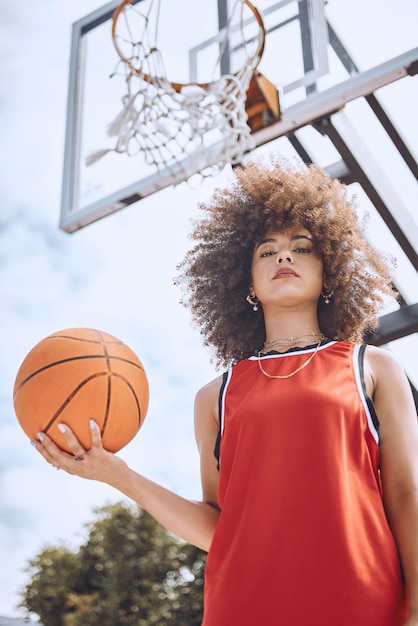In this vibrant photograph taken from a low angle, a young woman with light brown skin stands beneath a partially frayed basketball hoop. She is wearing a red sleeveless basketball jersey, trimmed with white and black around the neck and armholes. Her right hand is confidently gripping an orange basketball, revealing her white-painted fingernails. Her curly afro-style hair frames her face, which is adorned with makeup and accessorized with gold hoop earrings featuring a small dangling piece. Several small gold chains gleam against her neck. Behind her, the clear blue sky contrasts with the green trees, creating a dynamic outdoor setting. The photo, taken in daylight, conveys a strong, focused presence, capturing the essence of outdoor basketball against a scenic backdrop.